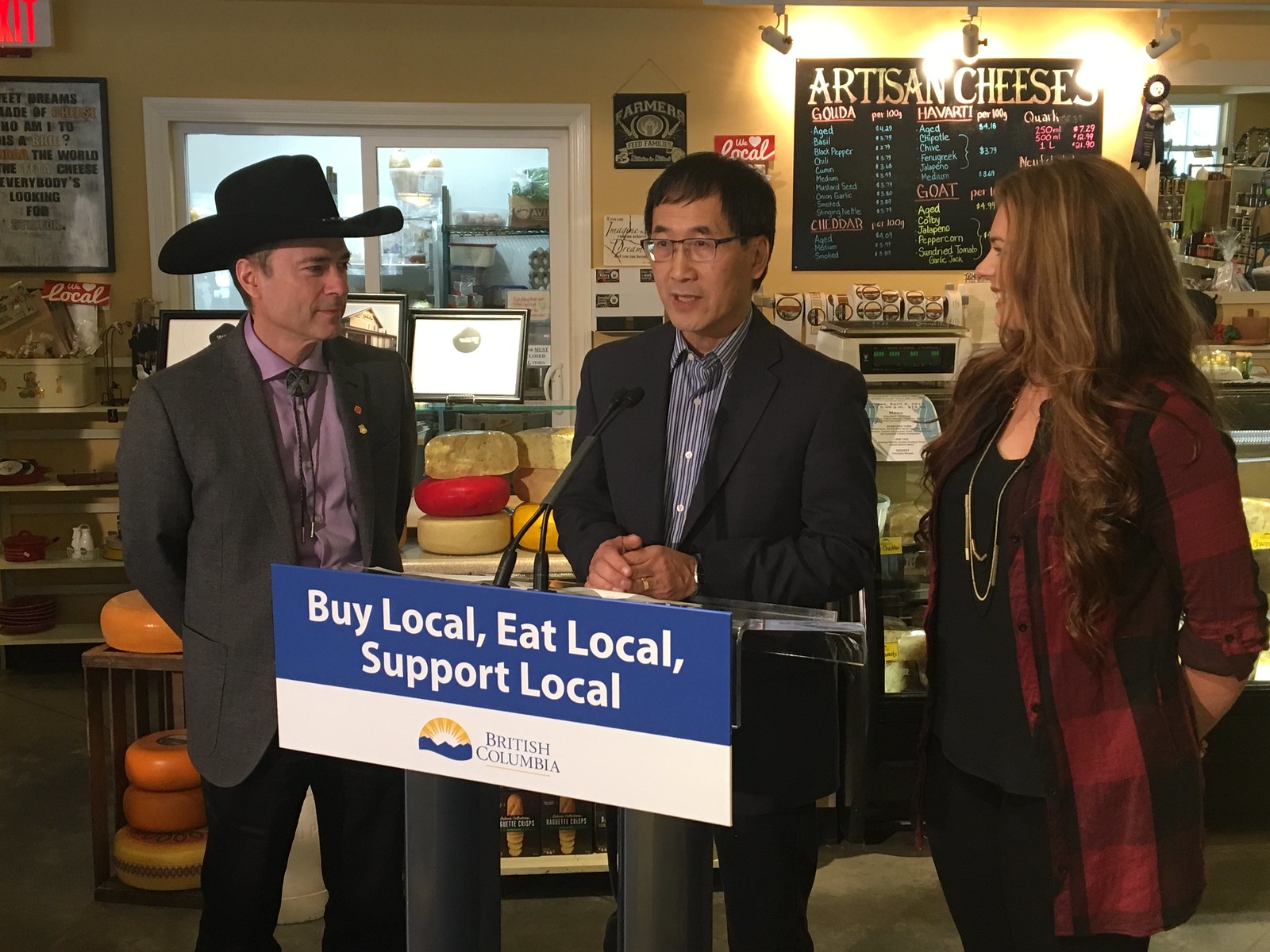The image depicts an Asian man in a navy blue suit and glasses, standing behind a podium that reads "Buy Local, Eat Local, Support Local, British Columbia". A microphone is affixed to the podium, which features blue and white text with the British Columbia insignia. To his left stands a woman in a red plaid dress with a coat over it, her hands behind her back, and to his right, a man in a cowboy hat, gray suit, purple dress shirt, bolero tie, and black jeans, also with his hands behind his back. The trio is positioned centrally in what appears to be a café or deli. Behind them, various signs and menu boards are visible, including one prominently displaying "Artisan Cheese". Glass display counters, typically used for meats and cheeses, and blocks of cheese add context to the market-like setting, which suggests an indoor environment during the day. The scene is vibrant with colors such as white, blue, and various shades of tan, red, orange, maroon, black, and purple.